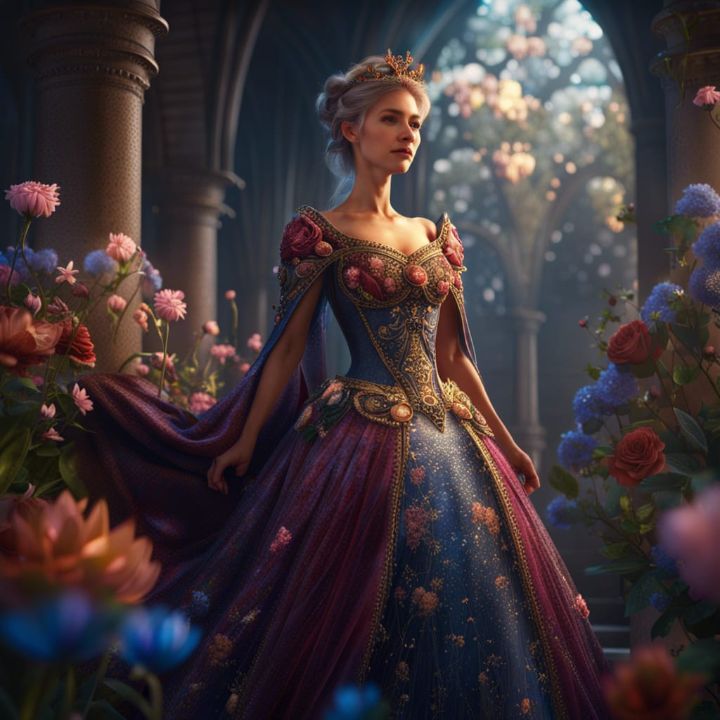The image depicts a fantastical, computer-generated scene likely inspired by digital animation, possibly resembling a Pixar movie environment. Set within a majestic castle, a queen or princess stands in a regal pose on a flower-lined walkway. The courtyard is brimming with vibrant blooms—red, pink, and blue—appearing both as clusters of roses to her right and as a variety of flowers including orchids to her left, some of which seem to catch on her flowing purple cape. Her ornate dress, primarily dark blue with pink floral embroidery, features gold filigree accents and a structured bodice resembling gold armor. A purple silk overlay complements her cape, and a gold belt cinches her waist. Her gray hair is elegantly styled up, crowned with a gold tiara. Light filters through flower-adorned windows in the background, enhancing the enchanting atmosphere of the scene.